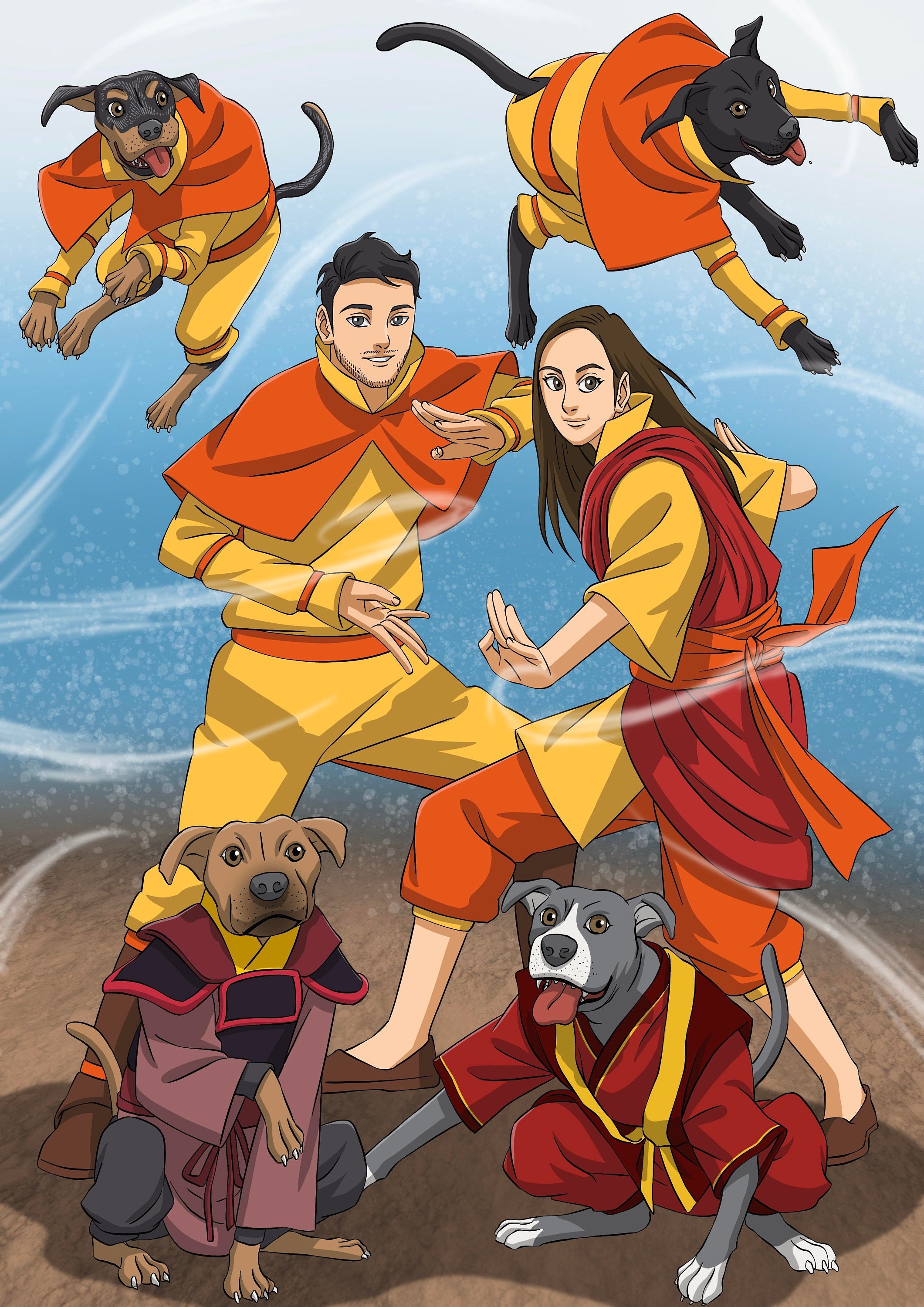A detailed animation in a rectangular portrait view showcases a vibrant scene featuring two people and four dogs. At the center, a man and a woman stand prominently, both adorned in colorful yellow and orange suits. The woman is additionally distinguished by a vivid red wrap. In the upper section of the animation, two dogs capture attention as they fly in mid-air; the one on the right is entirely black, while the one on the left sports a black and brown coat. Both airborne dogs are dressed in suits that match their respective fur colors.

At the bottom of the animation, two more dogs are positioned. The dog on the left has a light brown coat, and the dog on the right is gray and white. These ground-bound dogs also wear outfits, adding to the coordinated and lively aesthetic. The backdrop features a harmonious blend of light blue, white, and brown hues, creating a visually appealing setting that complements the characters and their attire.